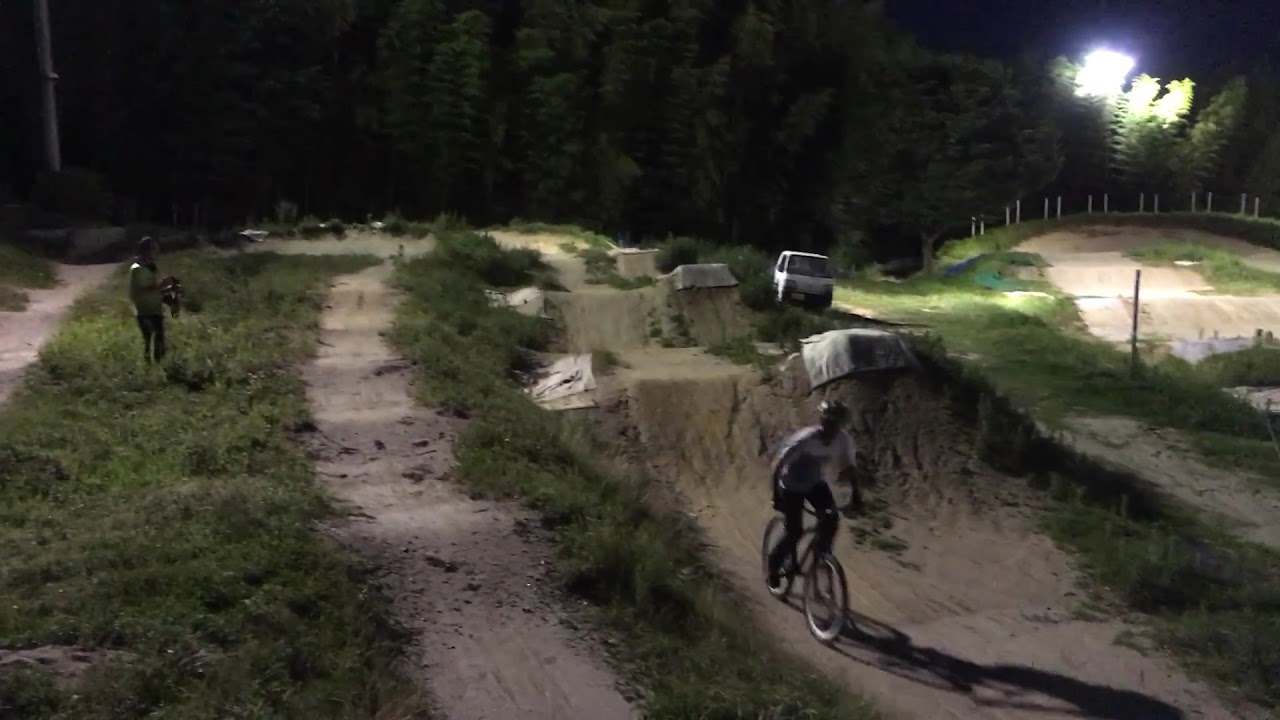The image captures a night scene on a BMX track situated in a dense forested area. In the lower foreground, a biker dressed in a white shirt, black pants, and a helmet is riding towards the camera. The track itself is composed of light tan or beige sand with patches of grass and weeds between the trails. On the left side, a person stands in the grass between two trails, possibly holding a camera. The far background is dominated by a grove of shadowy trees, and to the right, there are lights that might be reflecting off water, hinting at a body of water nearby or just additional lighting for the track. The scene is illuminated by artificial light whose source isn't visible in the image, creating a somewhat eerie and mysterious ambiance. Also in the background, there are faint and blurry outlines of what might be cars, along with some white fence posts and tan and gray rectangles on the ground, adding to the complexity of the setting.